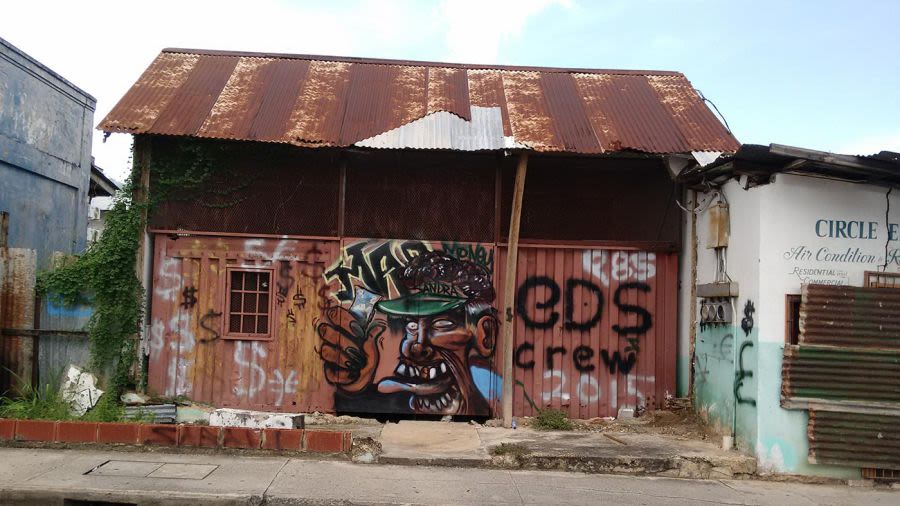In the image, an old, worn wooden building takes center stage, characterized by its heavily rusted tin roof which reveals patches of silver where the rust has chipped away. The structure is predominantly brown, with boarded-up windows using dark brown planks. The building showcases a vibrant array of graffiti, most notably a large caricature mural of a black man donning a green visor with a white brim. The man appears to be holding something in his hand and has an open mouth, while a heart on his head says "Sandra." Additional graffiti includes black and silver dollar signs, along with the inscription "CDS crew 2015." The left side of the building features a white wall with text advertising "Circle E, Air Condition, Residential, Commercial." The scene is framed by adjacent structures on either side, set against a backdrop of a light blue sky with scattered white clouds. In the foreground, a grey, concrete road enhances the rustic and weathered feel of the setting.